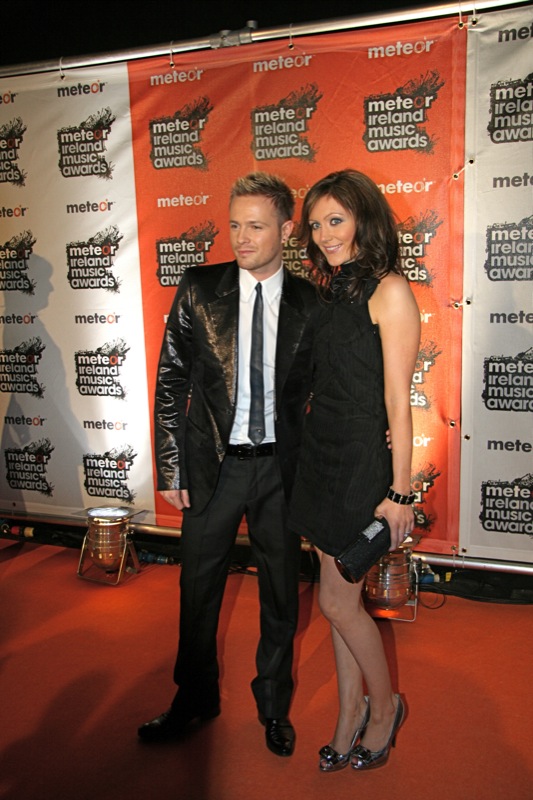In this photo, a man and woman, possibly celebrities or Irish musicians, are posing together on the red carpet at the Meteor Ireland Music Awards. The backdrop, a repetitively patterned banner with alternating white and orange sections displaying the event's logo, highlights the occasion. The man, positioned on the left, sports a dark black leather jacket over a white button-down shirt, paired with a thin black tie, black formal pants, and black dress shoes. His spiked, dirty blonde hair adds a touch of edginess to his look. To the right, the woman is striking in a short black dress and silver high-heeled shoes. She carries a clutch and has brown hair and blue eyes. The pair are smiling and looking off to the left, presumably at photographers capturing the moment.